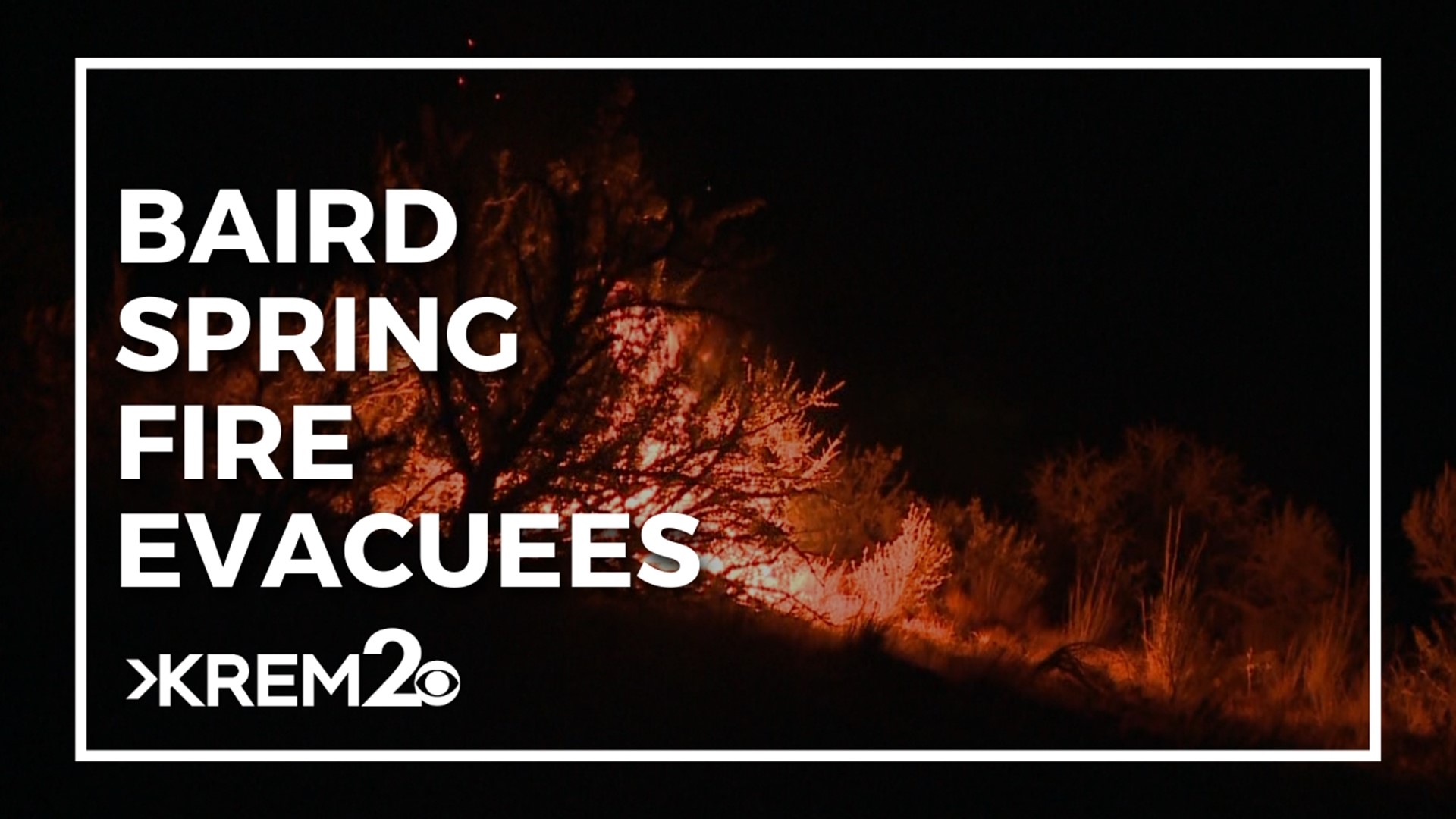In this nighttime rectangular image, a dramatic wildfire illuminates an otherwise dark scene. The photo's backdrop showcases a burning hill, with the highest part on the left, sloping downward to the right, enveloped in an orangey-red glow that highlights small trees, bushes, and grass. The inferno, set against a mostly black expanse, casts a fiery reflection off the silhouetted flora.

Positioned within the image is a prominent white border, inset slightly from the photo's edge. Overlaid on this frame are the words "Baird Spring Fire Evacuees," displayed in large, uppercase sans serif font along the left side. Below this, the text "KREM 2" and the CBSi logo identify the television station, suggesting that this image is part of a news coverage segment by a CBS affiliate. The visual composition and textual elements combine to convey the urgent and impactful nature of the event being reported.